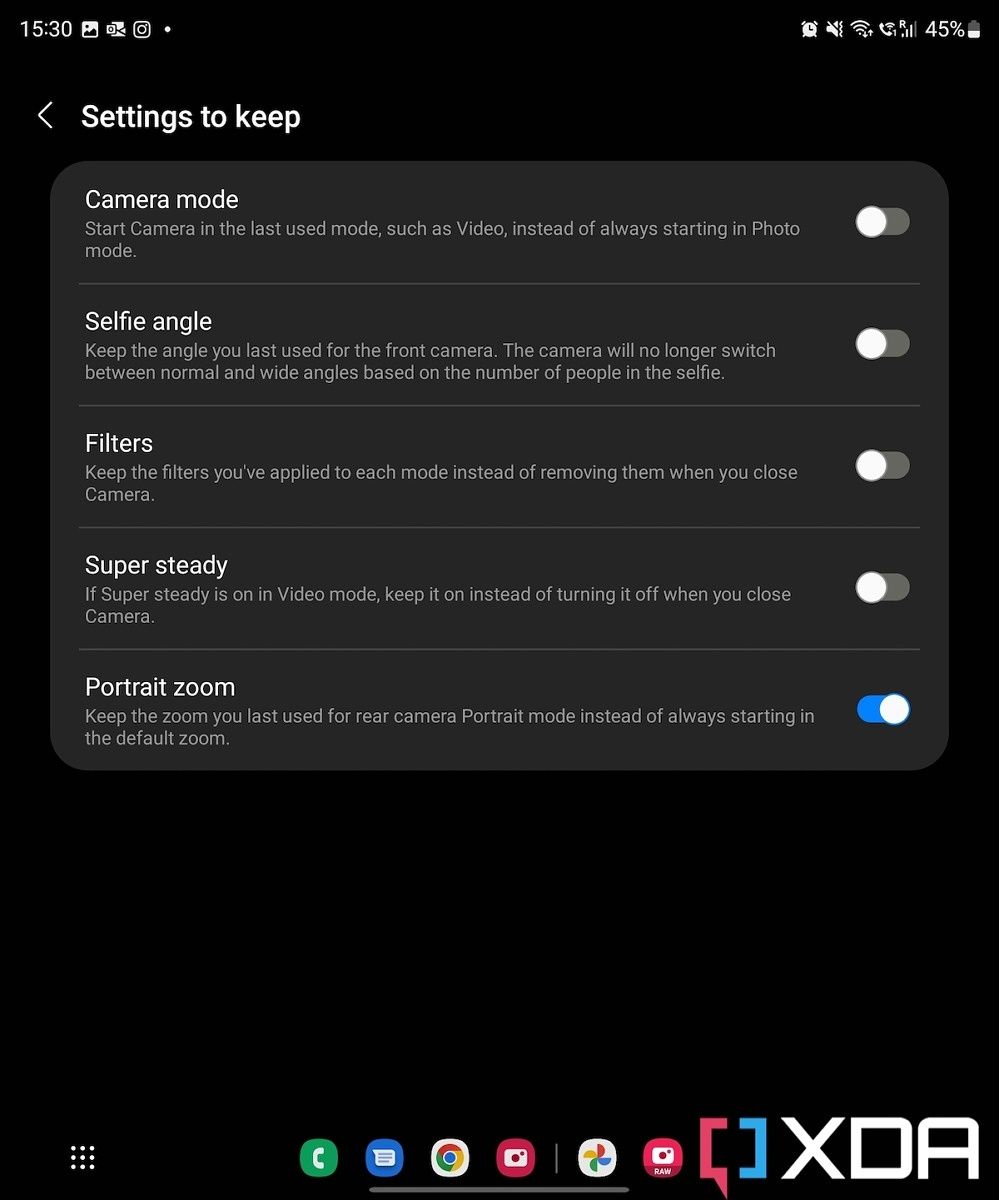This image appears to be a screenshot taken from the display of either a computer or a cell phone. At the top of the screen, the time reads 15:30. Alongside the time, various status icons are displayed, including a battery icon indicating that the battery life is at 45%. To the left, there is a back arrow, followed by the label "Settings to keep" in white text.

As you move down the screen, the first setting listed is "Camera mode," which is turned off. Below that, "Selfie angle" is also set to off. Both settings are displayed with a pill-shaped toggle switch, where the white circle on the left side signifies that these options are currently off. If these settings were on, the circle would be slid to the right.

Further down, the settings for "Filters" and "Super steady" are also shown, both in the off position. The last setting, "Portrait zoom," is the only one that is turned on, indicated by a blue-highlighted switch.

At the bottom of the screen, there are several icons that one can select or click. These icons include a square grid with dots, a phone, a speech bubble, and several others.

This detailed screenshot highlights the specific settings and their statuses, providing a clear visual representation of the user interface.